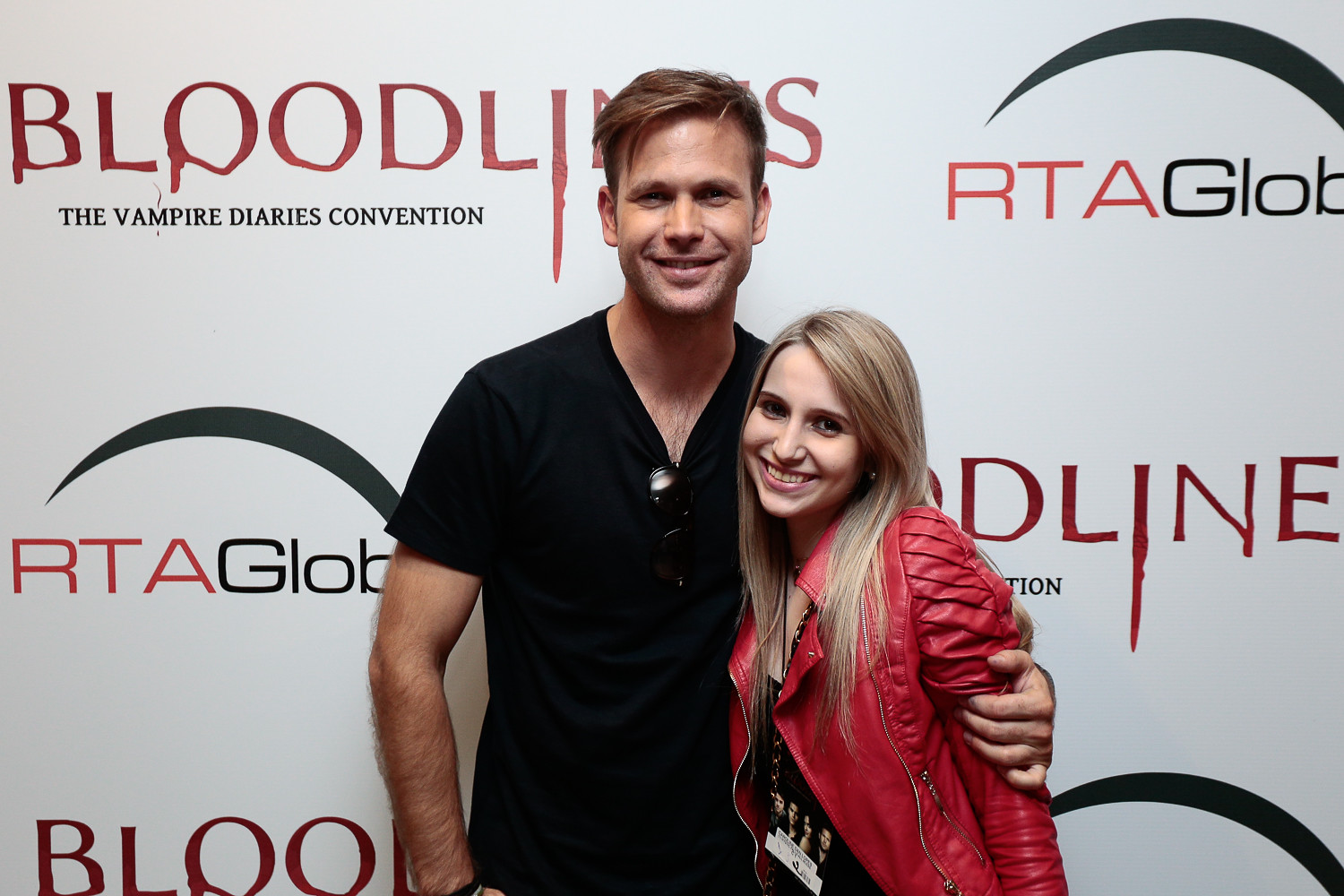In this indoor photograph, we see a joyous moment captured between two individuals at the Bloodlines, the Vampire Diaries Convention. The taller individual, a middle-aged man with short brown hair, stands on the left. He is smiling warmly at the camera, wearing a black short-sleeve shirt with sunglasses casually hanging from its collar. His arm is wrapped around a young woman who appears to be a devoted fan. She is petite, with long blond hair, and she beams at the camera, clearly thrilled to be there. She is dressed in a vibrant red leather jacket over a black shirt, and she wears a lanyard around her neck that features images of TV show characters, likely from The Vampire Diaries. Behind them, the convention's signage reads "Bloodlines, the Vampire Diaries Convention" with additional text that likely says "RTA Global," part of which is partially obscured. This setting, along with the evident excitement and shared smiles, suggests a meet-and-greet scenario, possibly a red carpet event, underscoring the fan-celebrity dynamic.